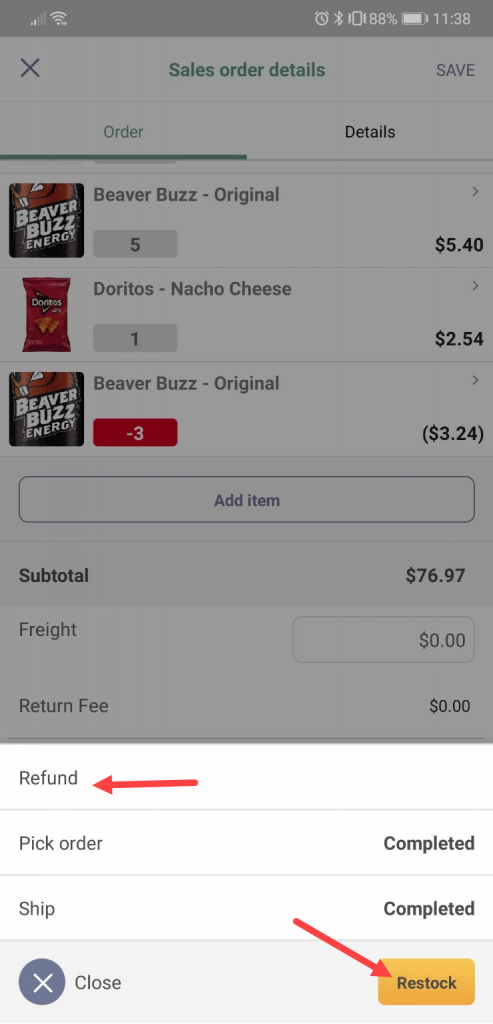This screenshot, taken from a phone, showcases the interface of a sales order management application. At the top of the screen is a grayed-out banner, containing several icons on the right side, including an 88% battery indicator and the time displayed as 11:38. Below this banner, bold letters prominently display "Sales Order Details," with an "X" on the left for closing the window, and "SAVE" in all caps on the right.

The interface is divided into multiple sections. The first section features tabs labeled "Order" and "Details," with "Order" highlighted, indicating the current page view. Under this section, the first item listed is "Beaver Buzz Original," represented with a product icon and a quantity of 5 in a rectangle. The price is indicated as $5.40, followed by a directional arrow pointing to the right.

The next line item, "Doritos Nacho Cheese," includes a product image of a Doritos bag, a quantity of 1, and a price of $2.54. Below this, a return entry for "Beaver Buzz Original" shows a quantity of -3 in a red rectangle, indicating a credit of $3.24.

Further down, a large rectangle labeled "Add Items" invites users to include additional products. In bold text, the "Subtotal" is displayed as $76.97, with accompanying details such as "Freight" ($0) and "Return Fee" ($0) listed below in regular font.

At the bottom of the screen, options for processing the order are provided, including "Refund" accompanied by a red arrow, "Pick Order Completed," "Ship Completed," and "Close" featuring an "X." Finally, a diagonal red arrow points to "Restock" inside a yellow rectangle, indicating the option to restock returned items.